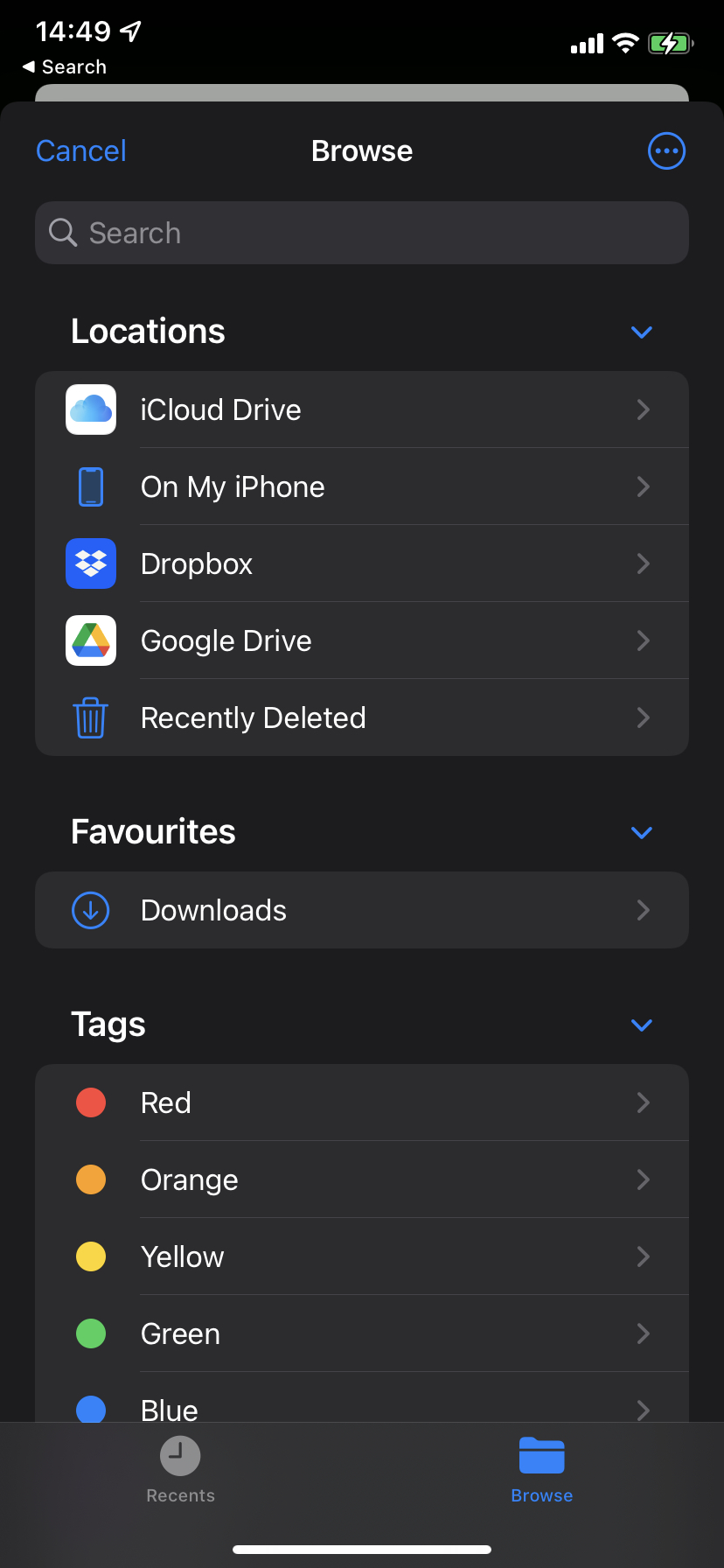The image depicts a smartphone screen showcasing a file management application. The status bar at the top displays the time as 14:49 along with icons for cellular signal strength and Wi-Fi connectivity. Below the status bar, there's a navigation section featuring a back arrow labeled "Search" in white and a blue "Cancel" button on the right.

Central to the screen is a header with the word "Browse" in the middle, accompanied by a blue circle containing three vertical dots, signifying additional options. Directly beneath this header is a search box for locating specific files or folders.

The primary content area of the screen includes a "Locations" menu with a dropdown list offering several storage locations: iCloud Drive, On My iPhone, Dropbox, Google Drive, and Recently Deleted. Below the locations, a "Favorites" section presents a "Downloads" tab for easy access to commonly used files. 

At the bottom of the list, there's a "Tags" section, displaying color-coded tags with labels for organizing files by colors: Red, Orange, Yellow, Green, and Blue. 

The footer of the screen has a navigation bar with two tabs: "Recents" and "Browse," with the "Browse" tab highlighted and featuring a folder icon. The interface primarily uses white text on a gray background, making the various options and file management features easily readable. This setup facilitates the organization of files into different folders and supports cloud storage solutions for efficient file management.